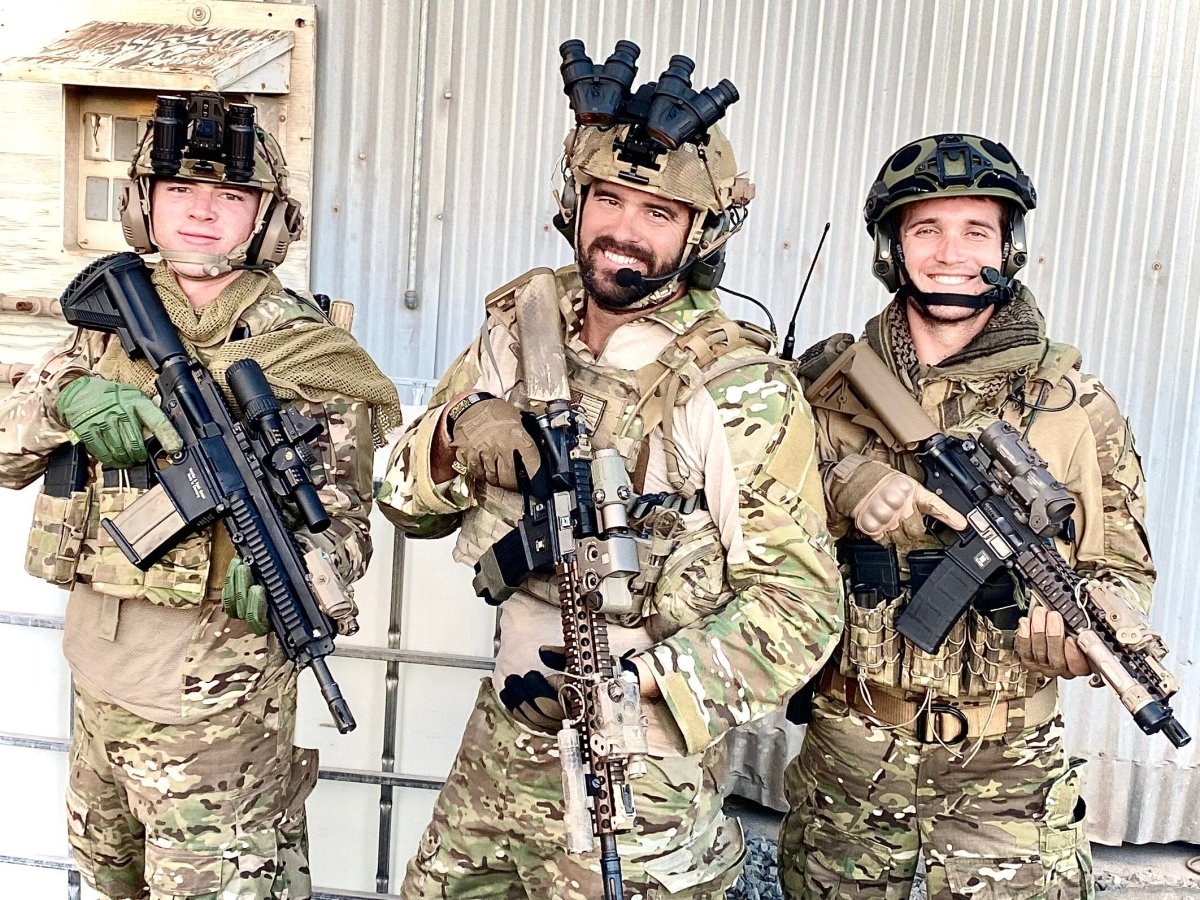This photograph captures three soldiers standing against a textured, tan-colored wall with vertical lines, indicative of a corrugated metal or vinyl siding building. All three soldiers are dressed in desert camouflage uniforms comprised of tans, greens, whites, and blacks. Each of the men is equipped with a helmet, gloves, and a firearm, and they are all smiling at the camera, signaling a moment of camaraderie.

On the far left, the soldier has fair skin and a slight smile. He is distinguished by his green gloves, black gun held downward, and binoculars mounted on his helmet. His helmet includes an additional piece of gear, possibly a lighting device.

The central figure appears to be the oldest among them, with a dark beard and a broad, open-mouth smile. He wears a tan helmet equipped with two pairs of binoculars. This soldier holds a tan-colored gun downwards and wears tan gloves, and his helmet also hosts additional equipment, perhaps used for lighting or nighttime operation.

On the right stands another smiling soldier with fair skin. He sports a black and tan helmet, holds his gun similarly downward, and wears tan gloves. Behind them, to the left, is a window covered by some sort of shielding, possibly a plywood awning or a cloth cover. The overall atmosphere is one of light-heartedness and unity among the soldiers.